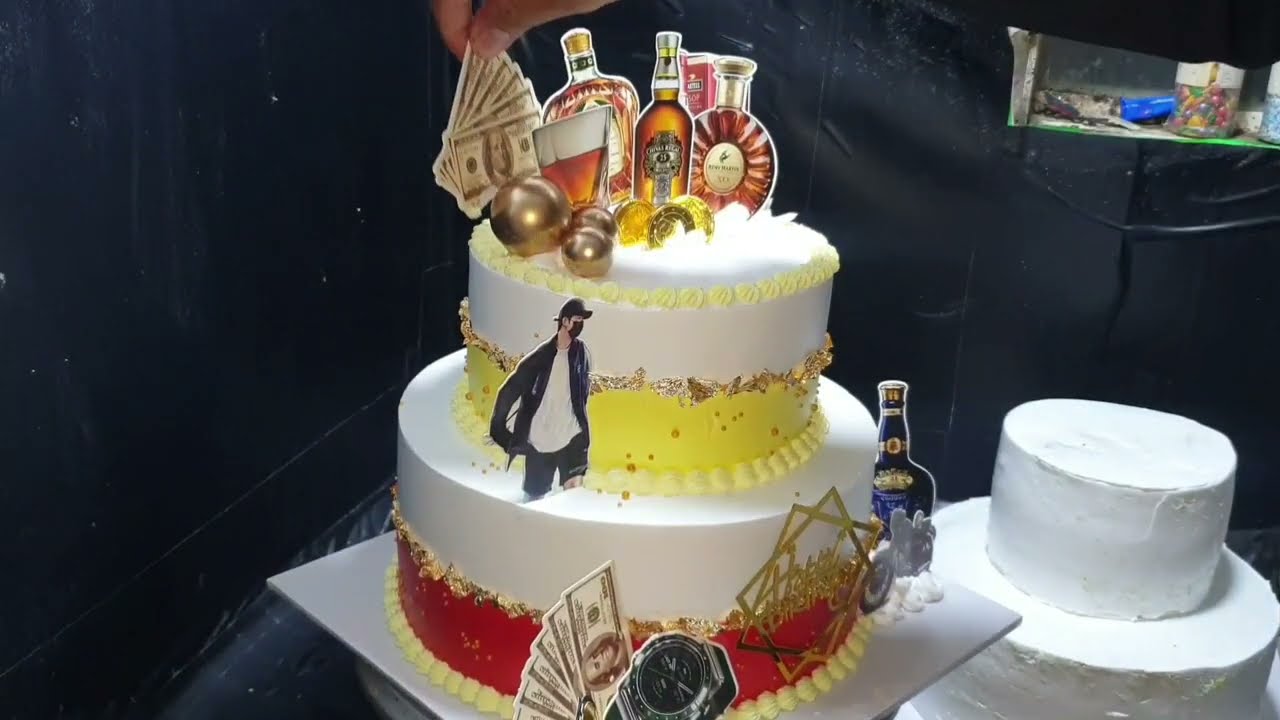The image captures a lively and detailed scene featuring two cakes displayed prominently on a table. The focal point is a two-tiered white cake with red and yellow-gold trimmings, adorned with a variety of intricate decorations. At the top, there is a character figurine dressed in a black jacket, white shirt, and black hat, wearing a mask. Surrounding the figure are paper cutouts of various ornate liquor bottles and a partially filled shot glass. Additional elements include scattered dollar bills, a wristwatch, a larger gold ball flanked by two smaller ones, and several gold coins, possibly accompanied by a gold ring. To the right of this elaborate cake, there’s a simpler, undecorated white cake. The background features black fabric draped behind the table, hinting at an indoor celebration, likely a bachelor party. In the distance, a container filled with multicolored balls adds a touch of vibrant color to the setting. The image is rich with hues including black, white, yellow, red, gold, brown, and blue.